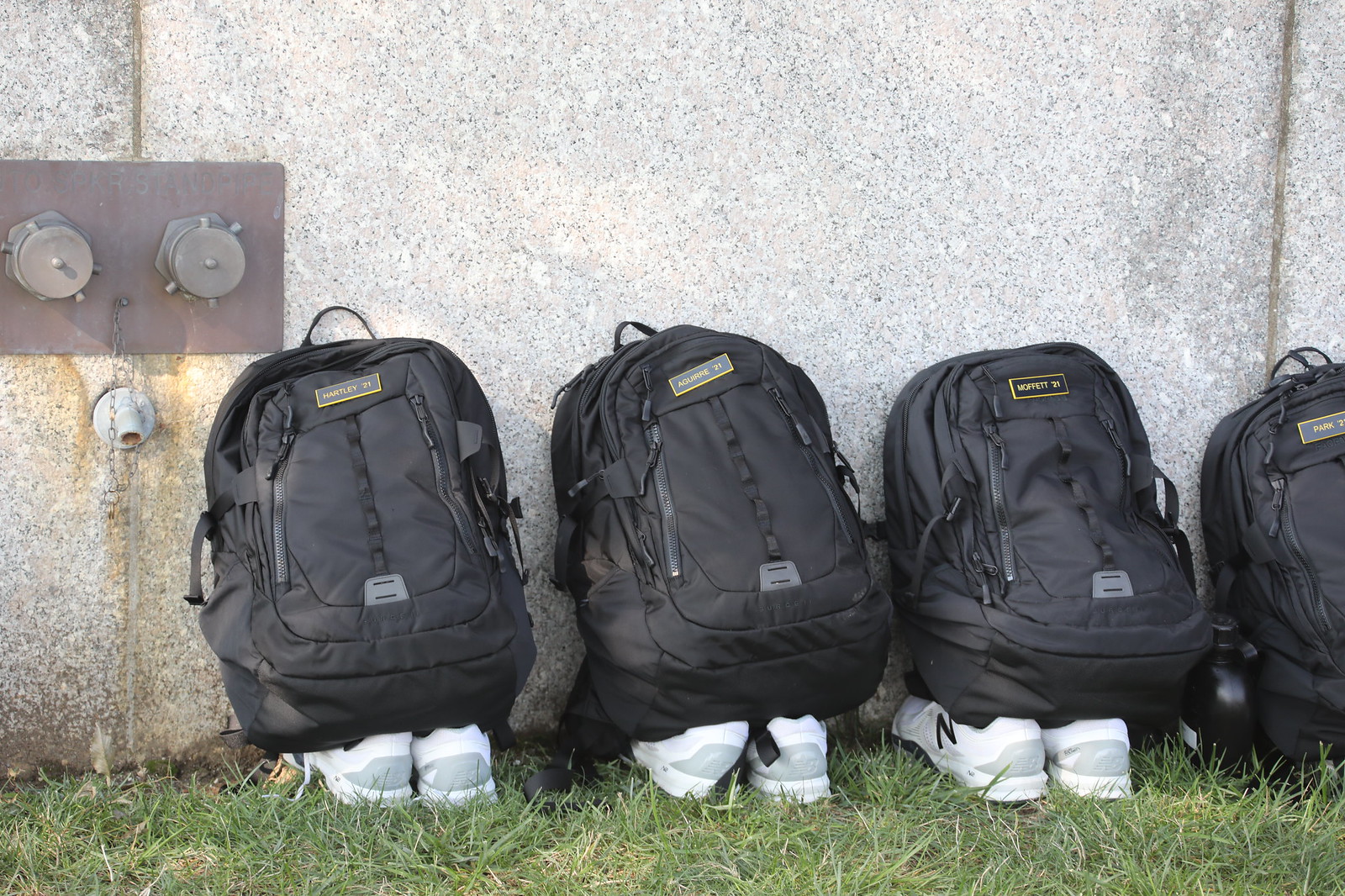The image depicts four identical black backpacks, each adorned with a black and gold label at the top, lined up against an outdoor speckled cement wall. Three of the backpacks are fully visible, sitting directly on white New Balance running shoes, identifiable by the black "N" logo. The fourth backpack is partially cut off on the right side of the image, but likely also rests on a pair of shoes. The ground beneath the backpacks and shoes is grassy. To the left of the image, there is a metal plate affixed to the wall, featuring two cylindrical objects and a small faucet below them.